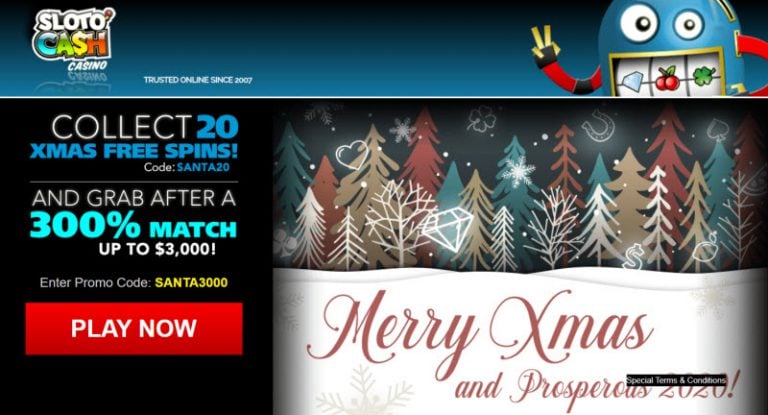The image is a promotional banner from the Slotto Cash Casino website, which has been a trusted online platform since 2007. The top portion prominently features the Slotto Cash Casino logo, followed by the tagline "trusted online since 2007." Below this, an animated character resembling a slot machine robot is displayed, designed to evoke the imagery of aligning three cherries in a slot game. 

Further down, the banner entices users with a special offer, stating, “Collect 20 Xmas Free Spins” with the promotional code "Santa 20." Below a faint gray line, it continues to advertise another exclusive deal: “Grab a 3000% match up to $3,000” using the promo code "Santa 3000." A bold red button with white uppercase text urges users to "PLAY NOW."

To the side, the banner wishes visitors a "Merry Christmas and prosperous 2020," featuring festive elements such as Christmas trees, snowflakes, a diamond, and a beautifully decorated sky, enhancing the holiday spirit.